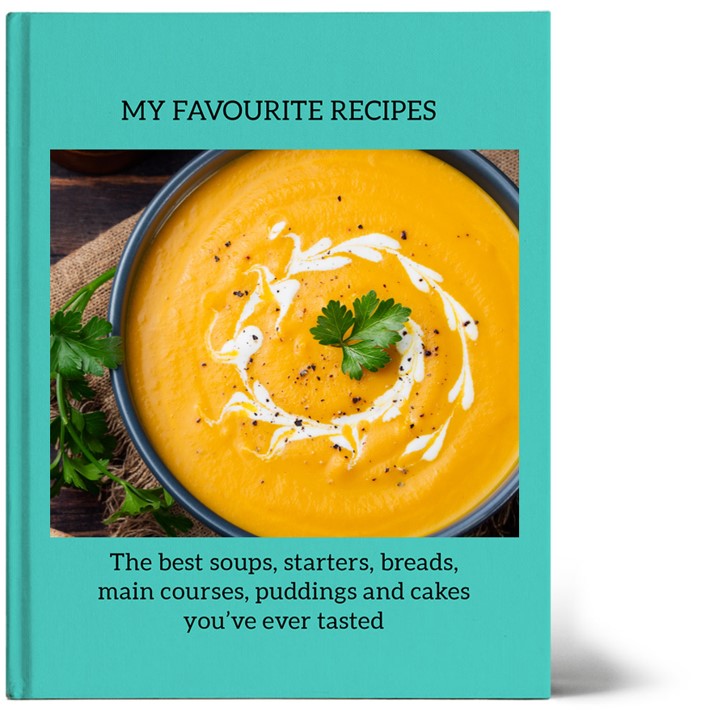The image depicts the cover of a book titled "My Favorite Recipes," prominently displayed in dark lettering at the top. The background color of the book is blue, and the spine is visible on the left side. Below the title, a large, vibrant image of a bowl of orange lentil soup is featured, adorned with swirls of white and bits of brown. A sprig of cilantro sits elegantly atop the soup as garnish. The bowl is blue, and a piece of burlap can be seen to its left with additional sprigs of green. The bottom of the cover, in black letters, promises "The best soups, starters, breads, main courses, puddings, and cakes you've ever tasted." The overall appearance of the book cover is clean and brightly lit, enhancing its inviting and appetizing presentation.